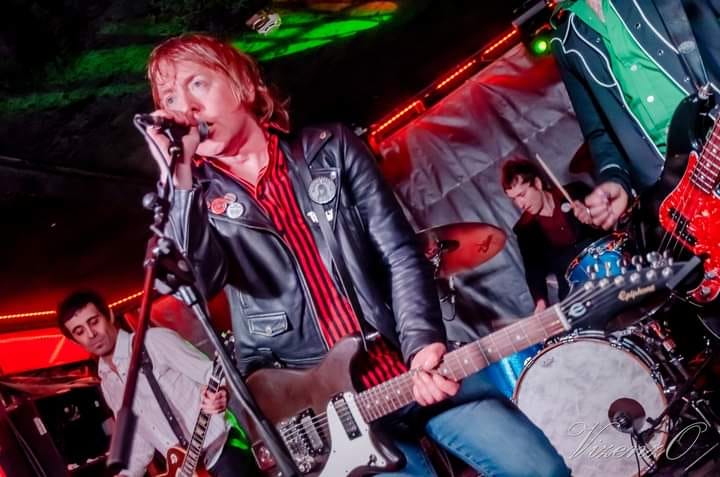In the image, a high-energy rock band is performing in a small, dimly-lit venue adorned with neon-like lights in shades of green, red, and orange. The central figure is the lead singer, who is also playing a brown and white electric guitar. He is distinctively dressed in a black biker jacket, red and white striped shirt, and jeans. To his left, another guitarist in a white shirt and possibly black pants plays a classic red guitar. In the background, the drummer, who is dressed in black with a red shirt and has black hair, is energetically playing his drum set. On the right, partially cut off from the photo, is the bassist in a green shirt and navy blue jacket, playing a black and red bass guitar. The venue's ambiance is accentuated by orange neon lights and intermittent strobe effects against a predominantly black backdrop.